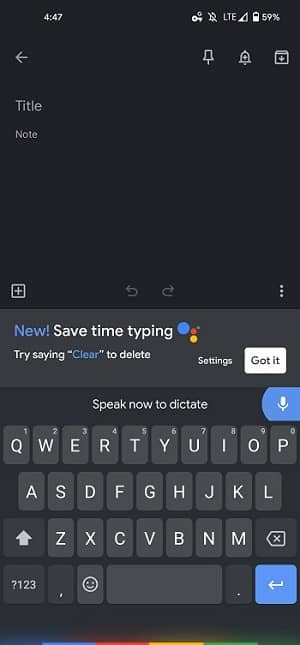Screenshot of a Mobile App with Time-Saving Typing Feature:

The screenshot showcases a mobile app on a black screen, displaying a time-saving typing feature. At the top left, the time reads 4:47. In the top right corner, there are six icons: a notification bell with a line through it, LTE signal indicator, a triangle denoting reception strength, a battery icon showing 59% capacity, and numerics confirming 59% battery capacity.

Below this row, a gray left arrow is on the left, with three icons on the right: a thumbtack, a notification bell, and a file folder. Beneath this is a blank square section labeled with "Title" and "Note."

At the bottom of the screen, four icons are present: a plus sign on the left, forward and backward arrows in the center, and three vertical dots on the right. Centrally displayed in blue text is "New!" followed by "Save time typing." It also includes a suggestion: "Try saying 'clear' to delete." To the right, there are "Settings" and a clickable white "Got it" pill bar.

Below this, a line reads "Speak now to dictate," accompanied by a blue pill bar with a microphone icon. Finally, there is a keyboard layout at the bottom. The top row starts with Q and ends with P: Q-W-E-R-T-Y-U-I-O-P. The second row contains: A-S-D-F-G-H-J-K-L. The third row has an up arrow, followed by Z-X-C-V-B-N-M, and a delete button. The lowest line includes: a question mark/number toggle, emoji icon, spacebar, period, and a blue enter arrow.